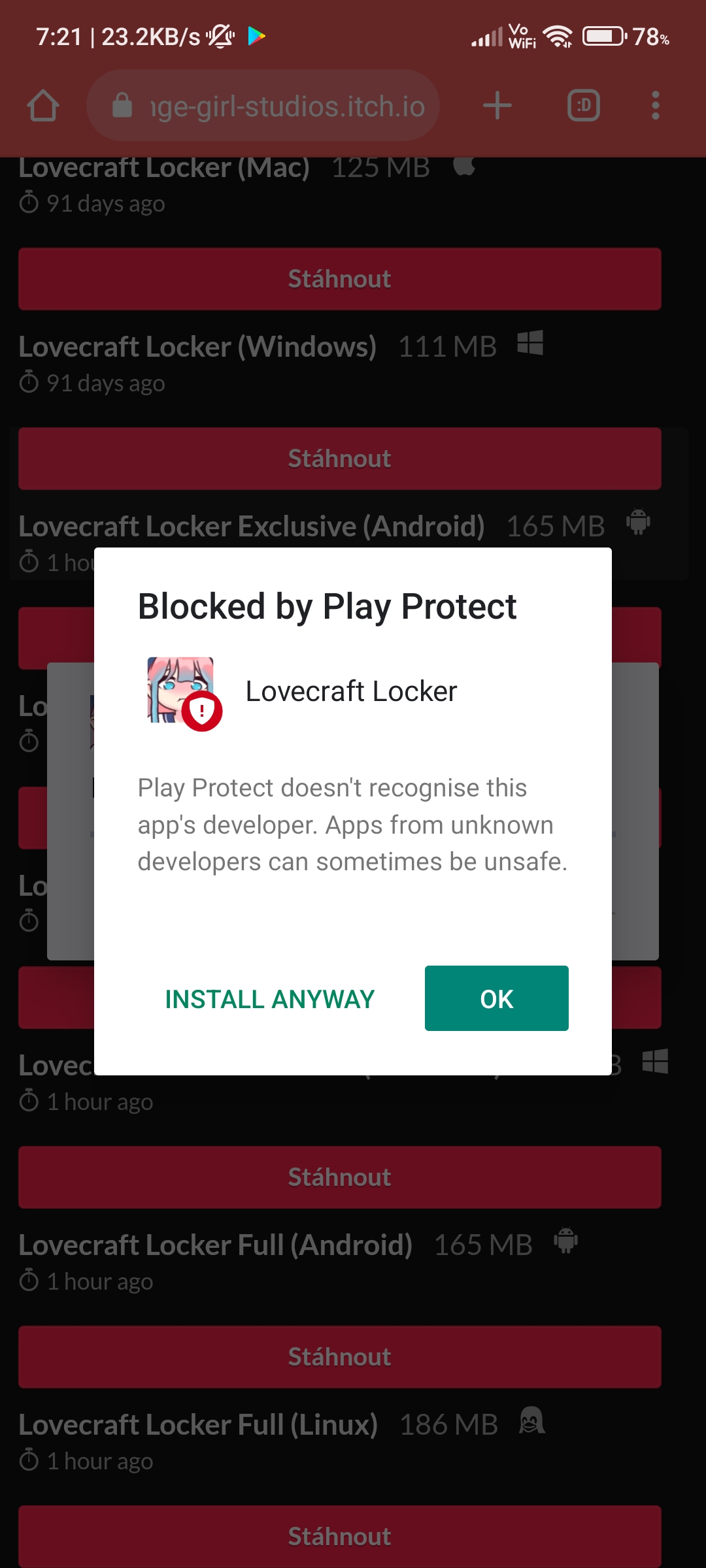The image shows a screenshot from a phone. At the top, the status bar displays various icons and information. On the left, it reads "721," separated by a thin white line from "23.2," which is likely kilobytes. Next to this is a bell icon with a slash through it, indicating silent mode, and a play icon. On the right, there is a signal bar showing three full bars, a Wi-Fi icon, and a battery indicator at 70%. Beside the battery icon, there is a house icon, a search area, and a circle icon.

Below the status bar is the main content area. The background features the text "Lovecraft Locker" with "windows" in parentheses beneath it. A red bar runs underneath this title, extending down the page, overlapping the image. The text "Blocked by Play Protect" appears prominently along with "Lover Lock Lovecraft Locker."

There is also an image of a character within a circle that has a caution sign. Below this image, there is a paragraph of text, followed by an "Install Anyway" message and an "OK" button.